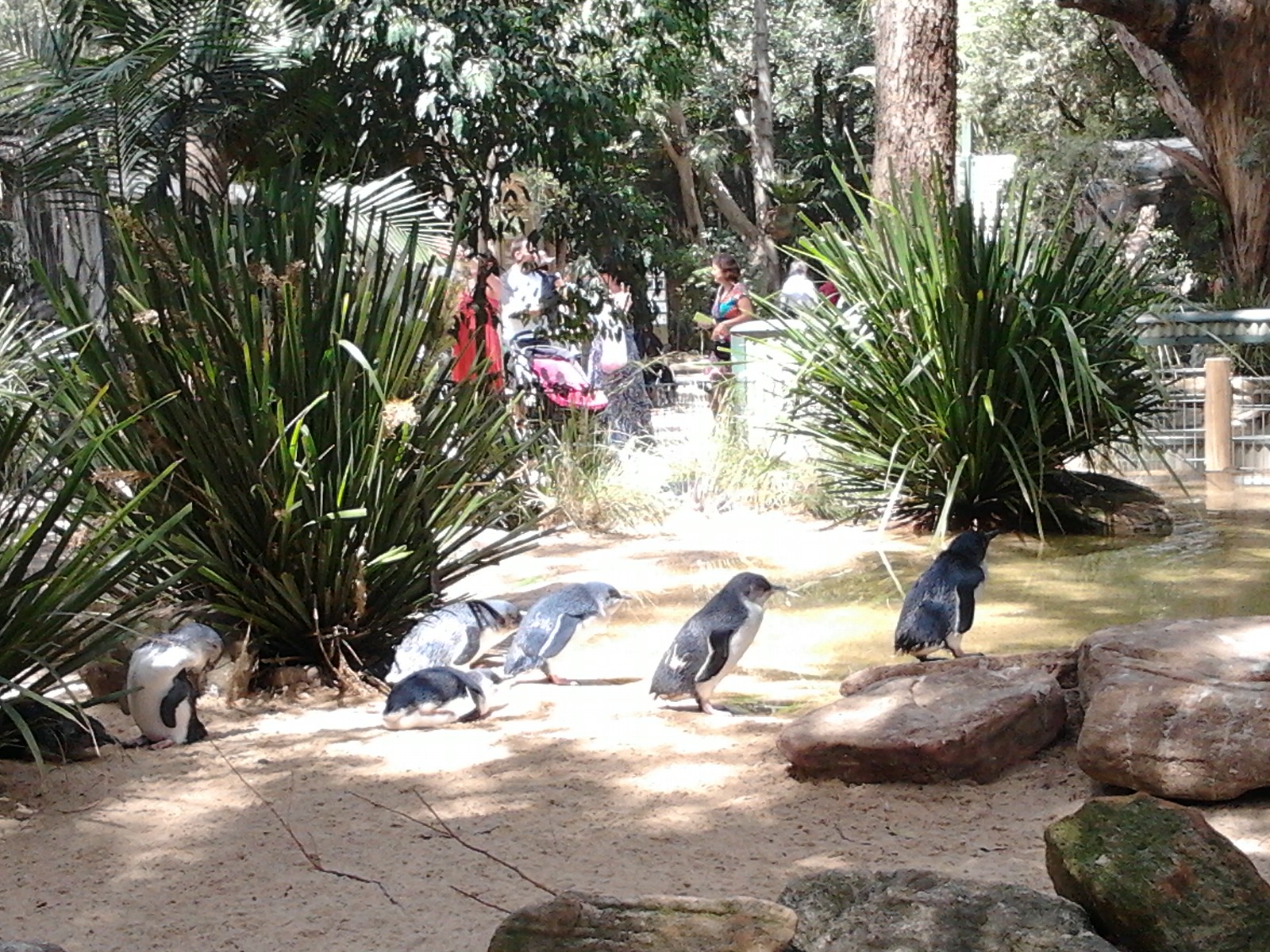This image captures a zoo exhibit featuring six small penguins, each about a foot to 18 inches tall, as they navigate a sandy, rocky ground that is speckled with black spots and scattered with broken branches. One penguin stands on a large flat rock located at the bottom right corner, while the others wander the sand. The surrounding exhibit includes patches of green leafy bushes and trees with tall, straight leaves, some of which are drooping. To the right, a small body of water is visible, enhancing the naturalistic setting of the enclosure. In the background, there is a fence that demarcates the exhibit, beyond which blurry figures of zoo visitors, including a woman in a colorful top, a woman in red, and another person with a baby cart, can be discerned. The far background reveals tall trees with lush, tropical foliage, contributing to the warm, vibrant ambiance of the scene.